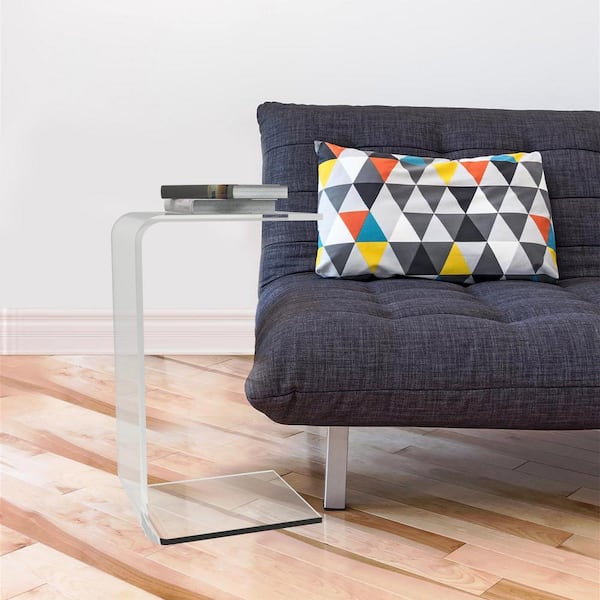The image depicts a minimalist living room setting featuring a stylish, clear plastic C-shaped end table strategically positioned next to a dark navy, denim-like futon. The table's design allows its base to slide seamlessly under the couch, making it convenient to pull over for a makeshift work surface. On this transparent resin table, two books are neatly placed, emphasizing its primary function as an end table. Surrounding the scene is a hardwood floor with a light wood stain and a diagonal layout that adds a modern touch. Against a backdrop of white walls with light peach-colored molding, the futon stands out with its plush cushions, evoking a sense of comfort. A distinctive rectangular pillow with a multi-colored triangle pattern, including shades of black, white, grey, yellow, blue, and orange, complements the overall contemporary and functional aesthetic.